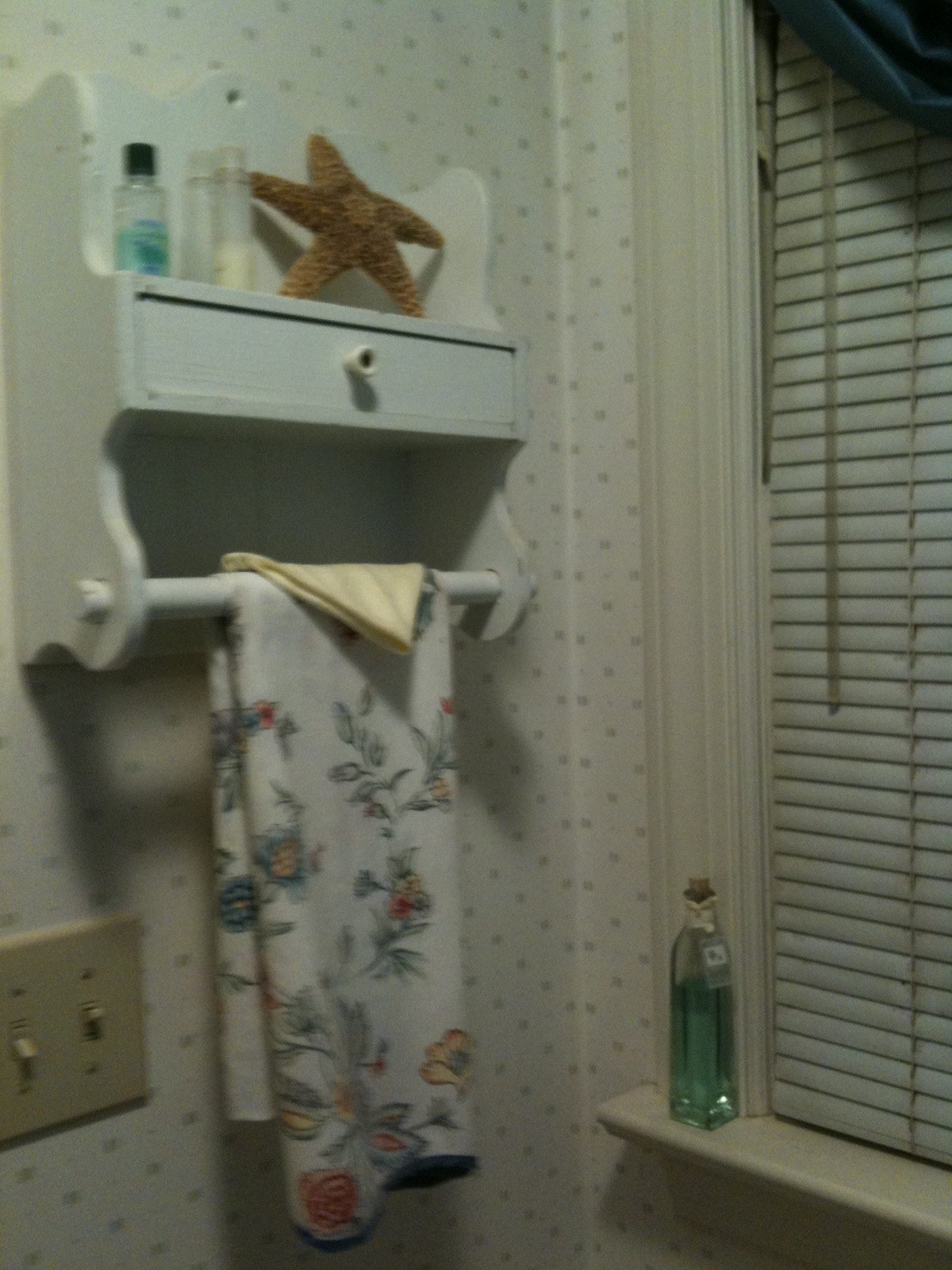The image captures a vintage corner of a bathroom, likely from the 1980s or 1990s. The bathroom's walls are adorned with white wallpaper featuring a small, subtle design. A windowsill, painted in an off-white, creamy shade, is framed by crown molding. The window boasts blinds that are pulled shut, with a curtain—perhaps in a midnight bloom pattern—pulled to the side, showcasing its creases and wrinkles.

On the windowsill, there's a bottle with a cork, adding to the nostalgic ambiance. To the left of the window, an older white shelving unit is mounted on the wallpapered wall. This shelf has a distinct character with curved edges on the back panel and is equipped with a small knob, indicating a drawer. The lower section of this shelving unit features a rod with a towel draped over it and another yellow item folded on top.

The top shelf of the unit displays decorative elements, including a starfish and a few bottles. Adjacent to the shelving and near the towel hangs a yellowish, cream-colored light switch, blending seamlessly with the vintage decor of the bathroom.